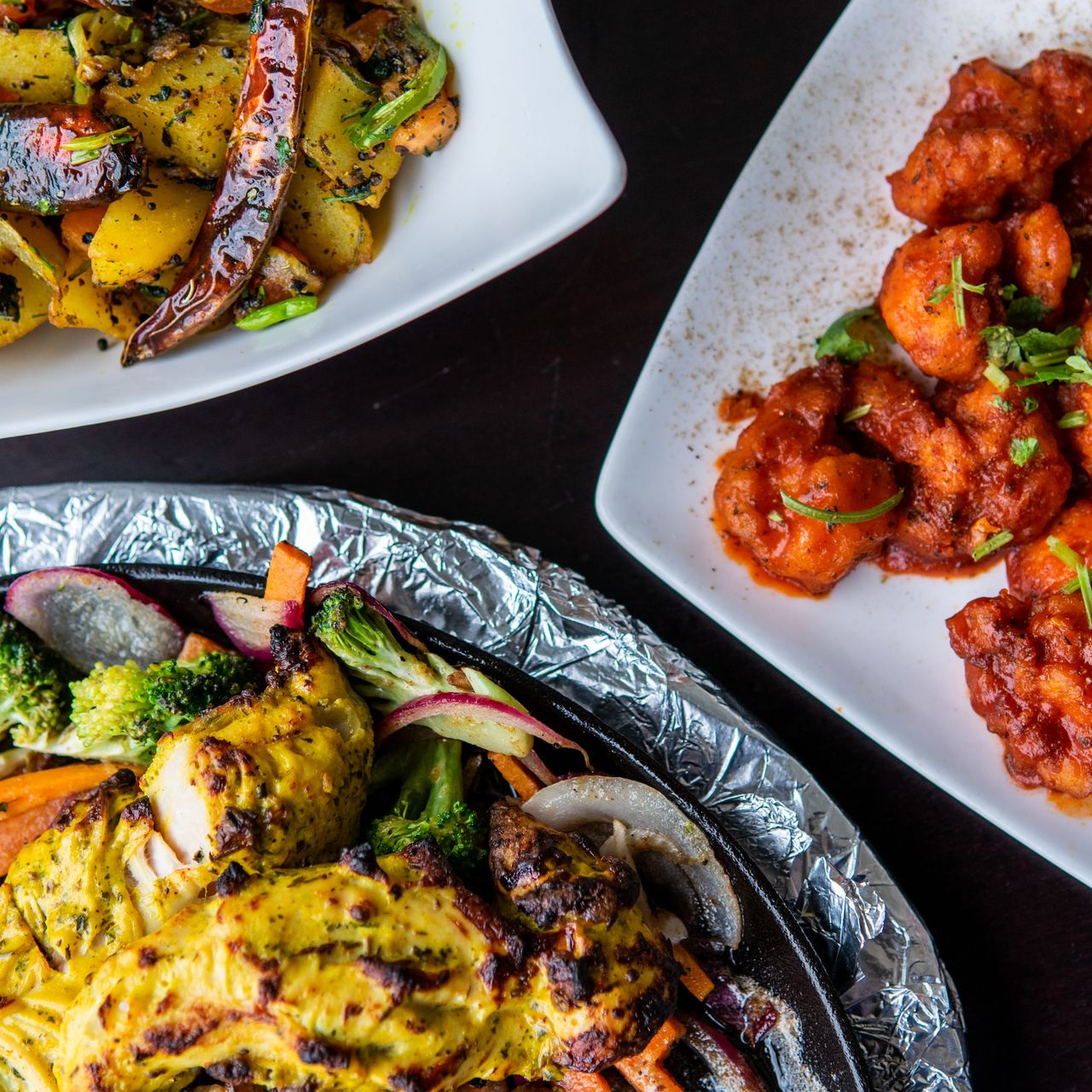The image showcases a selection of beautifully plated dishes, likely from a restaurant. The dishes are presented on two glass white plates, placed on a black surface. On the top left, there is a square plate featuring seasoned, fried potatoes, along with various vegetables like peppers and broccoli, which are garnished with green herbs. This plate also contains meat that could be either chicken or cauliflower, enveloped in an orange-red sauce and topped with green chives. On the bottom left, another dish is plated with chicken in a yellowish sauce, surrounded by grilled vegetables including broccoli, artichokes, radishes, and red and yellow onions. This dish appears partially wrapped in tinfoil. The vibrant array of food items is accented with seasonings and garnishes, making the presentation visually appealing.